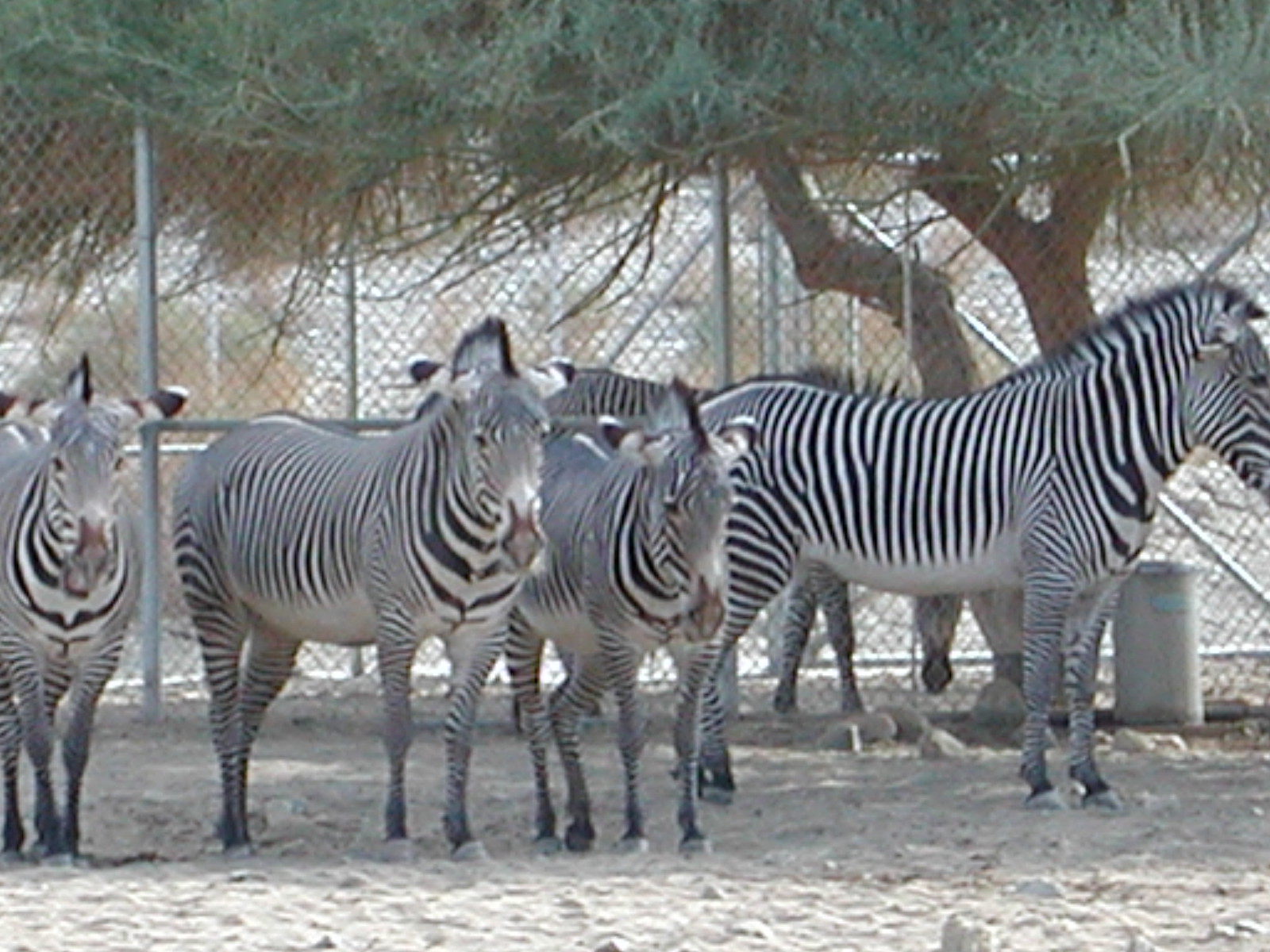This image depicts five zebras in a zoo-like enclosure with a sandy, dusty ground. Four zebras stand side by side in the foreground, all facing to the right. Three of these zebras, likely juveniles, are calmly positioned towards the left, while an adult zebra is seen in profile on the right edge of the frame. Partial visibility of a fifth zebra is noted from its mane and additional legs beneath the foreground zebras. The enclosure is defined by a tall chain-link fence extending across the background, securing the animals within. A large tree with a green leafy canopy casts a shadow over the zebras, providing some shade. Additional details include another tree partially inside and outside the cage on the far right and a trash can visible on the right side behind the zebras, enhancing the sense of a contained, managed environment.